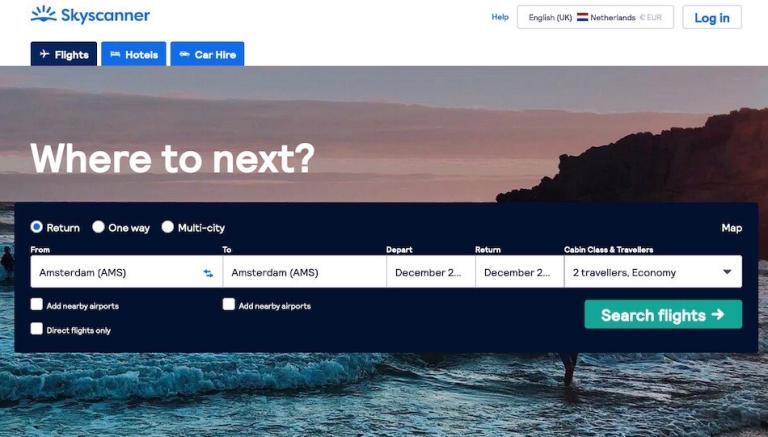At the top of the image, the word "Skyscanner" is prominently displayed in blue. Toward the right, the smaller text "Help" is also visible. An informational search bar follows with the language set to "English" and "UK" in parentheses; next to it is "Netherlands." To the right of this search bar is a square icon offering the option to "Log In." 

Below this, on the left, there is a dark blue square featuring the word "Flights" alongside a small image of a white airplane. Adjacent to this is the word "Hotels" in a medium blue shade, followed by "Car Hire."

The prominent lower half of the image depicts a serene sky during sunset, painted in shades of pink. On the right, there are tall, brown rocks. Below these rocks, the ocean shows off blue and white waves, with a person standing in the water.

At the top center, the text "Where to Next?" sets the stage for the options below. These options include "Return," "One Way," and "Multi-City." The option "Return" is highlighted in a blue-filled box. The search parameters read: "From Amsterdam to Amsterdam, Depart December 2nd, Return December 2nd, Cabin Class: Economy, 2 Travelers." Finally, a green rectangle containing the text "Search Flights" with an arrow pointing to the right completes the image, suggesting the action to begin the flight search.